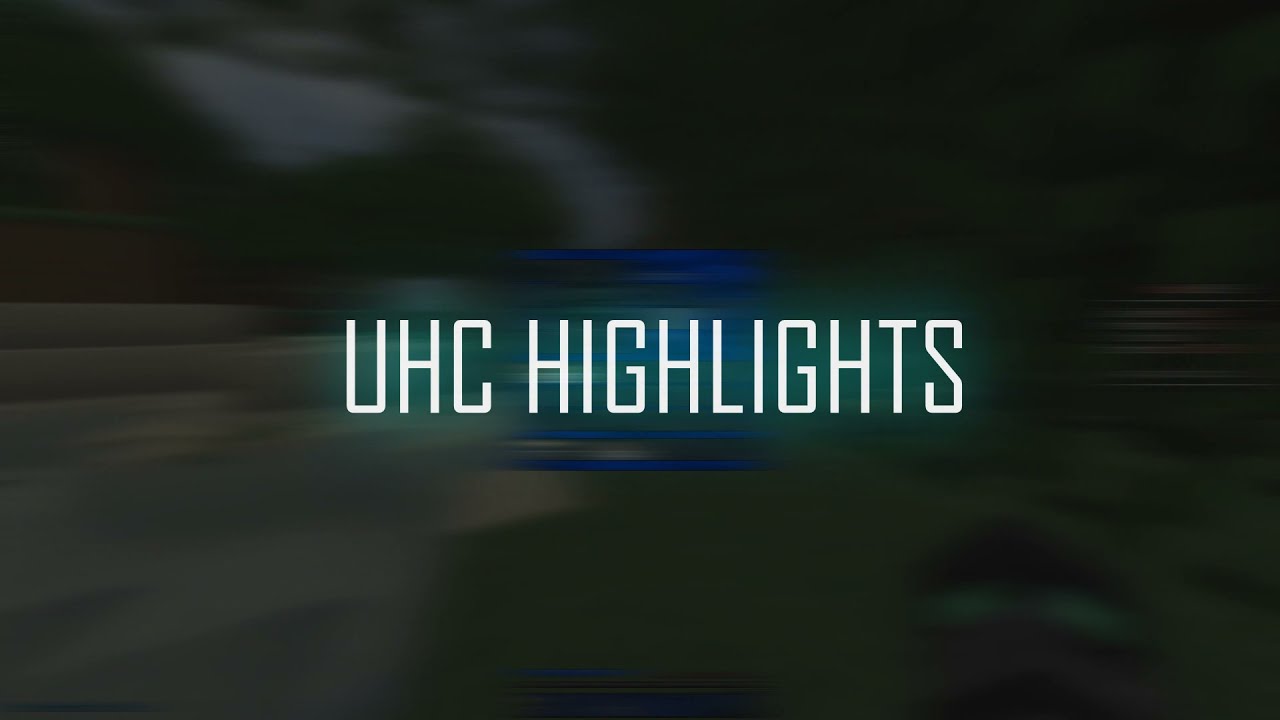The image appears to be a frame from a video or a banner, characterized by a predominantly black, underexposed background with indistinguishable features, suggesting motion blur or high-speed capture. Central to the image is the text "UHC Highlights," rendered in bold, block-like letters with a glowing greenish tint, emphasized by blue streaks both above and below the text. The background hints at an obscured and dark scene, possibly from video gameplay. On the left side, faint textures suggest sand or dirt, while on the right, there's an indistinct pair of lips or the first-person view of a hand, resembling elements from Minecraft. Despite the vague background, the focus on the clear, centrally positioned "UHC Highlights" text stands out prominently.